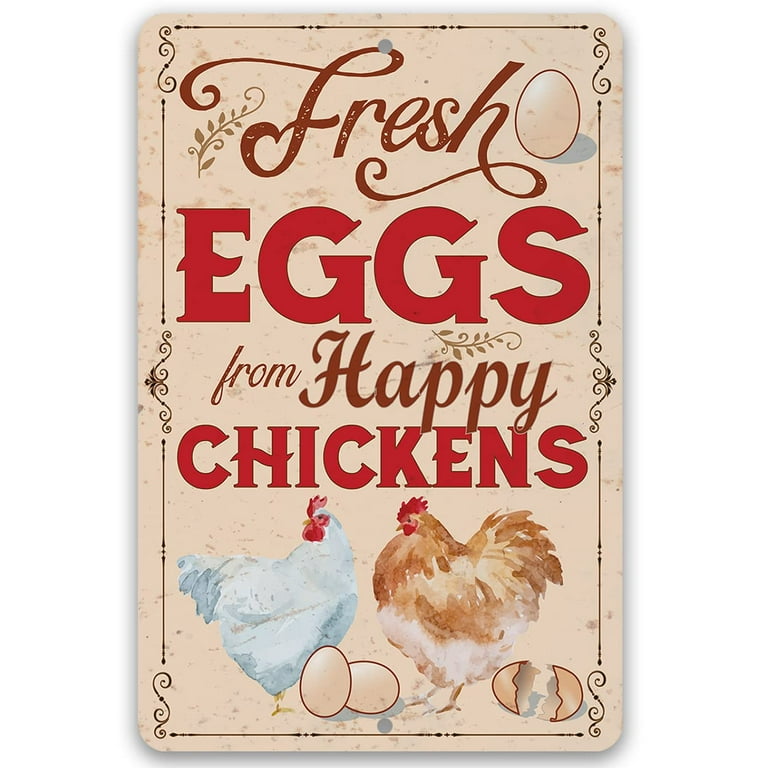The image is of a vintage-style poster set against a cream-colored background. The poster features an ornate black border with elegant scrollwork in the corners and center. At the top of the poster, a long leaf branch and an egg are depicted, alongside the word "Fresh" written in brown cursive. Below that, in large, bold red letters, it reads "EGGS." Further down, in brown cursive text, it says "FROM HAPPY," followed by "CHICKENS" in large, red block letters. At the bottom, two chickens are illustrated: a white chicken with a red comb and wattle facing left, and a brown chicken with a fuzzy white bottom, also with a red comb and wattle, facing the same direction. Between these chickens are two whole brown eggs and one cracked open egg showing its dark brown shell.